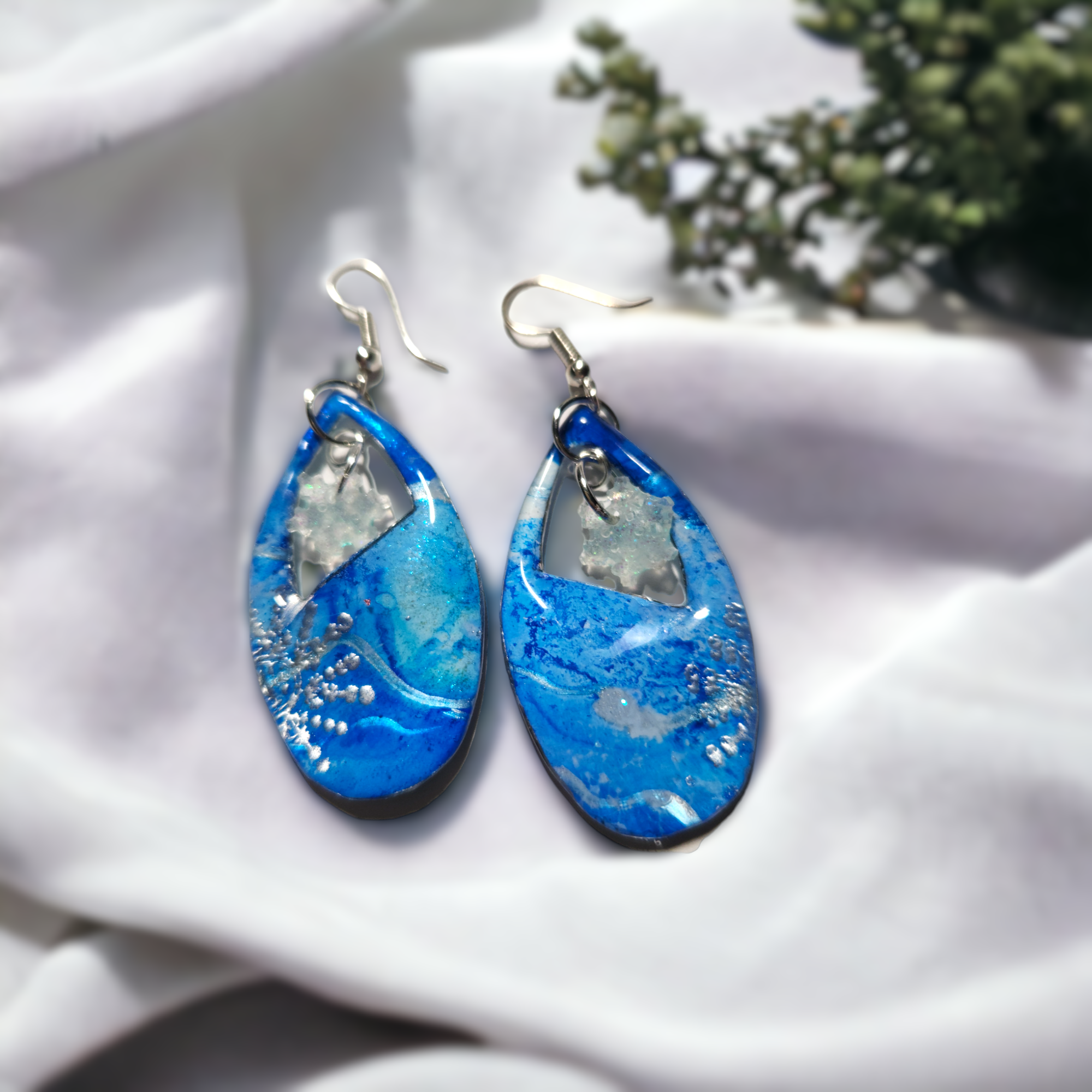This indoor photograph showcases a pair of exquisite, matching earrings that are artfully crafted from a material resembling resin or polymer clay. These teardrop-shaped earrings boast a mesmerizing tie-dye blue pattern, with varying intensities of blue that evoke the appearance of ocean waves or abstract art. Adorned with an embedded silver snowflake on one side, each earring also features a distinct teardrop-shaped cutout, presenting what appears to be a delicately carved white stone snowflake dangling at the center. 

The earrings are designed to dangle elegantly from silver hooks attached to delicate chains, promising a graceful look when worn. They are displayed against a soft, white fabric backdrop, which is likely a folded tablecloth or blanket, adding a textured contrast. In the background, there is an out-of-focus glimpse of greenery, suggesting a plant or tree, hinting at a cozy indoor setting with ample lighting, as evidenced by the soft shadows cast on the fabric. This detailed composition, with its blend of blue and silver hues, hints at a festive, possibly holiday-themed accessory.

---

(Note: The aim was to merge all the details while emphasizing on shared and repeated information for coherence and a detailed description.)